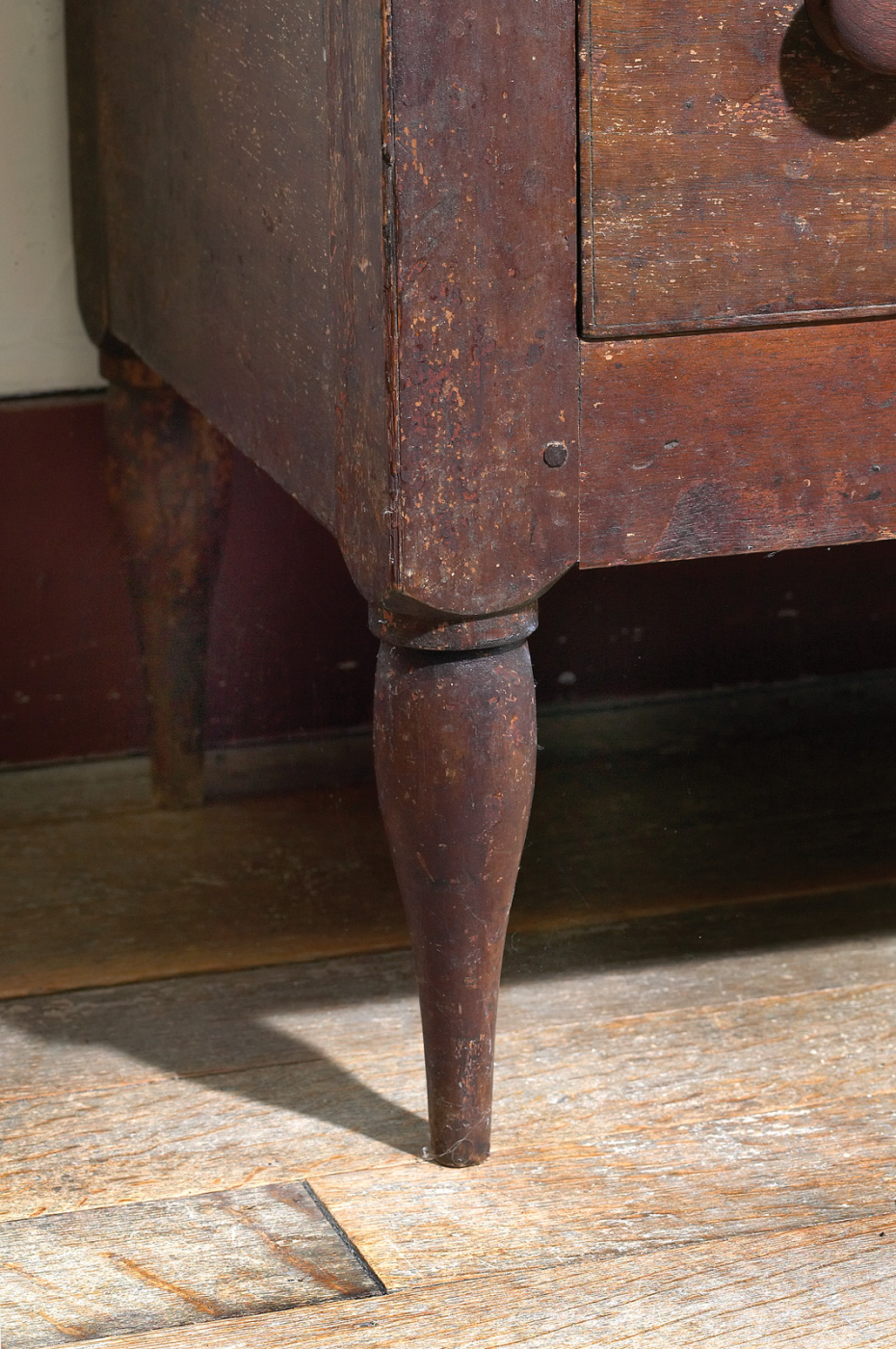This is a detailed zoomed-in, vertical rectangular color photo of an old wooden dresser, which is a rusty reddish brown color and shows considerable wear with numerous marks. The dresser's left front and left rear legs, each about six inches tall, are prominently displayed in the center and background of the image respectively. In the upper right-hand corner, a partial view of a drawer knob is visible, along with the bottom left-hand corner of the drawer itself. Shadows of the furniture are cast to the left of the image. The dresser is situated on an old, beat-up wood floor with a light brown, whitish color in a wooden design.